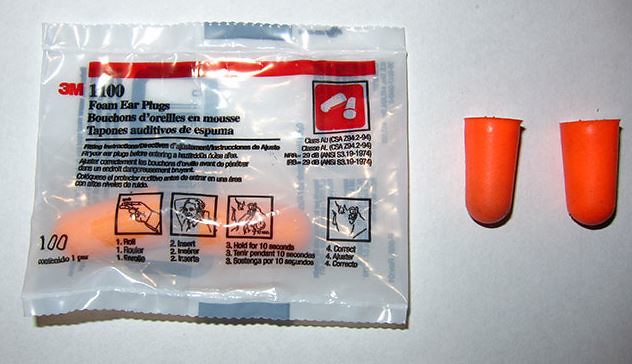This photograph depicts a pair of orange foam earplugs, both inside and outside their transparent plastic packaging, laid out on a white background under a light. The earplugs are shaped like cylinders with rounded bottoms, resembling thimbles or beakers. The packaging displays the 3M brand in red letters in the top left corner and includes various codes, as well as illustrated instructions for use in multiple languages. The term "tapons," the French word for earplugs, is also noted on the packaging.